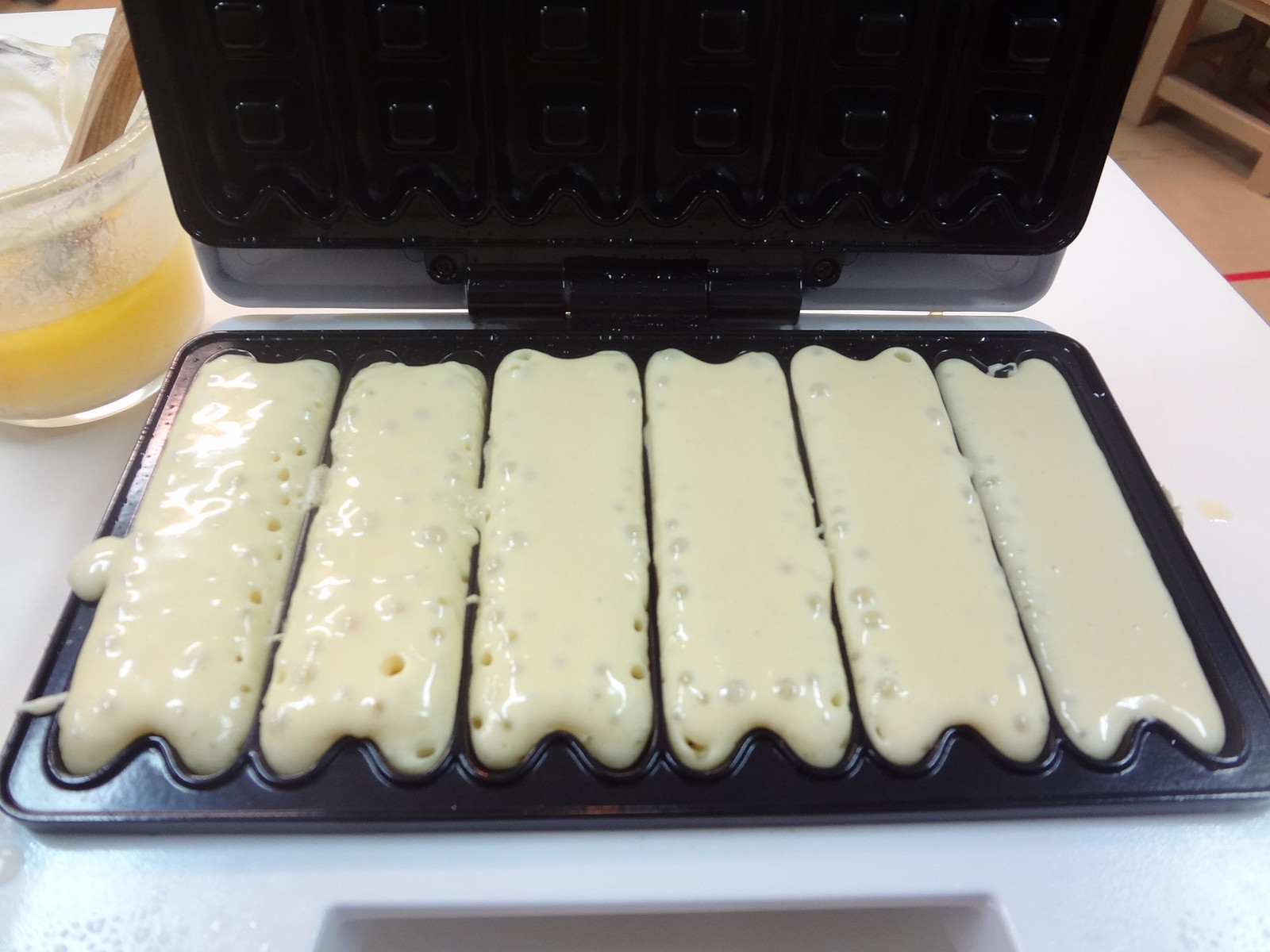This detailed photograph captures the process of making waffle sticks in an open waffle stick iron. The iron, which is black and resembles a grill, sits on a shiny white surface. The open lid reveals six vertical sections of pale batter, each filled nearly to the top and bubbling in anticipation of being cooked. The sections have wavy edges at both the top and bottom, and the top lid features a traditional waffle pattern. To the left of the waffle iron, there’s a clear, straight-sided cylindrical container with melted butter, into which a wooden-handled pastry brush is inserted. The container shows condensation from the warm butter. Additionally, there appears to be some liquid or oil present on the white surface, possibly from the baking process. On the front of the waffle iron is an opening that suggests a handle. The entire setup gives a sense of preparation and anticipation just before the waffle iron is closed to cook the batter into delicious stick-shaped waffles.